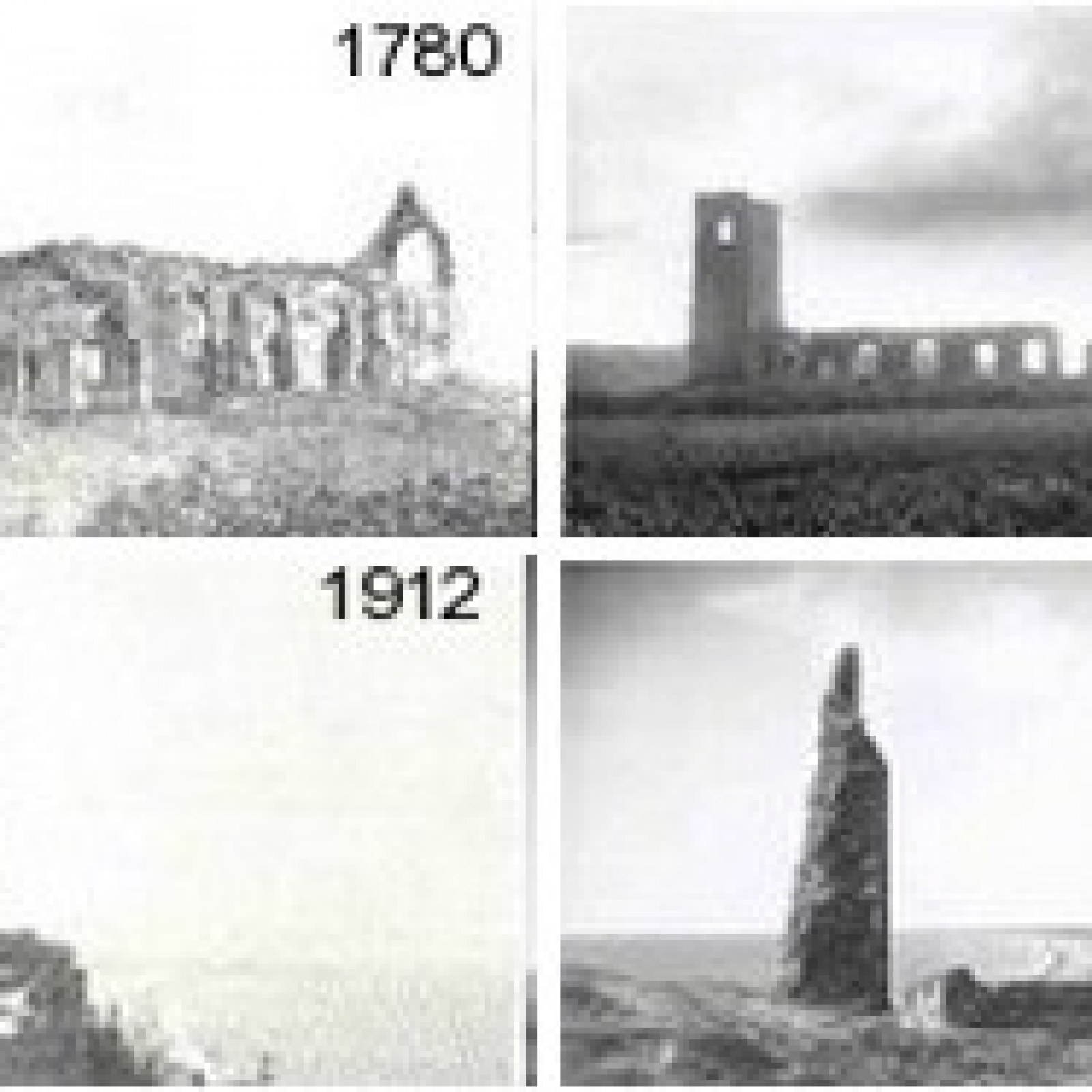This black and white collage features four grainy photographs, each depicting historical ruins. The top left image, labeled "1780" in black text, shows the dilapidated frame of an old church-like structure, evoking an air of decay and abandonment. In the top right image, we see a blurred, tall building with a courtyard, resembling an upside-down L-shape under a faintly visible sky. The bottom left photograph, marked "1912," presents a largely featureless, light gray expanse, save for a faint ghostly cutout, possibly remnants of a building's tower, suggesting further decay over time. Finally, the bottom right image captures a solitary monolith, standing vertically amidst the ruins, barely discernible through the film grain. The collage, with its progression from a tangible structure to near-oblivion, seems to depict the gradual disintegration of these historical edifices over time.